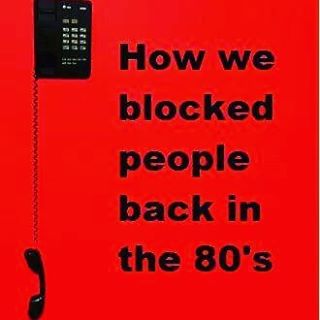The image showcases a digitally created, sentimental meme set against a bold red background. Dominating the scene is a vintage, black, wall-mounted push-button telephone with the receiver hanging down by its coiled cord, emphasizing its off-the-hook state. Complementing the visual, bold black text on the right side of the image humorously reads, "How we blocked people back in the 80s," capturing a nostalgic method of avoiding calls. The entire composition features a simple palette of blacks, whites, grays, and reds, contributing to its retro aesthetic.